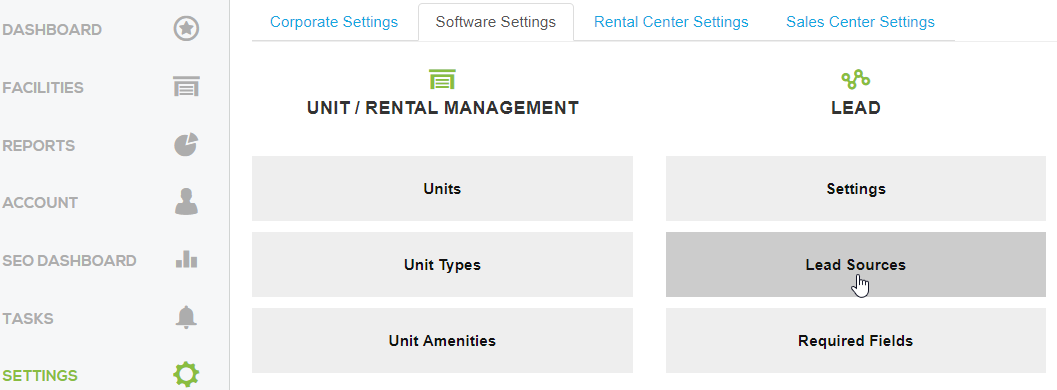The image showcases a comprehensive tool designed for rental and unit management tasks. On the left side, there is a vertical navigation menu featuring options such as Dashboard, Facilities, Reports, Accounts, SEO, Dashboard, Tasks, and Settings, with the Settings option highlighted in green while the rest remain in gray.

At the top right are horizontal tabs labeled Corporate Settings, Software Settings, Rental Center Settings, and Sales Center Settings. Software Settings is the selected tab, indicated by its black text, while the others are in blue. 

Beneath the tabs, the header reads "Unit / Rental Management." The area below this header is divided into sections with gray bars representing different categories. The first section includes bars labeled Unit, Unit Types, and Unit Amenities. 

To the right, there's another category labeled Leads, followed by three bars named Settings, Lead Sources, and Required Fields. The Lead Sources bar features a hand cursor pointing at it, suggesting it as a clickable link with a darker gray background, indicating its current selection.

Overall, this interface appears to be a powerful tool for managing various aspects of rental properties, from unit details to lead tracking and source management within the Software Settings area.